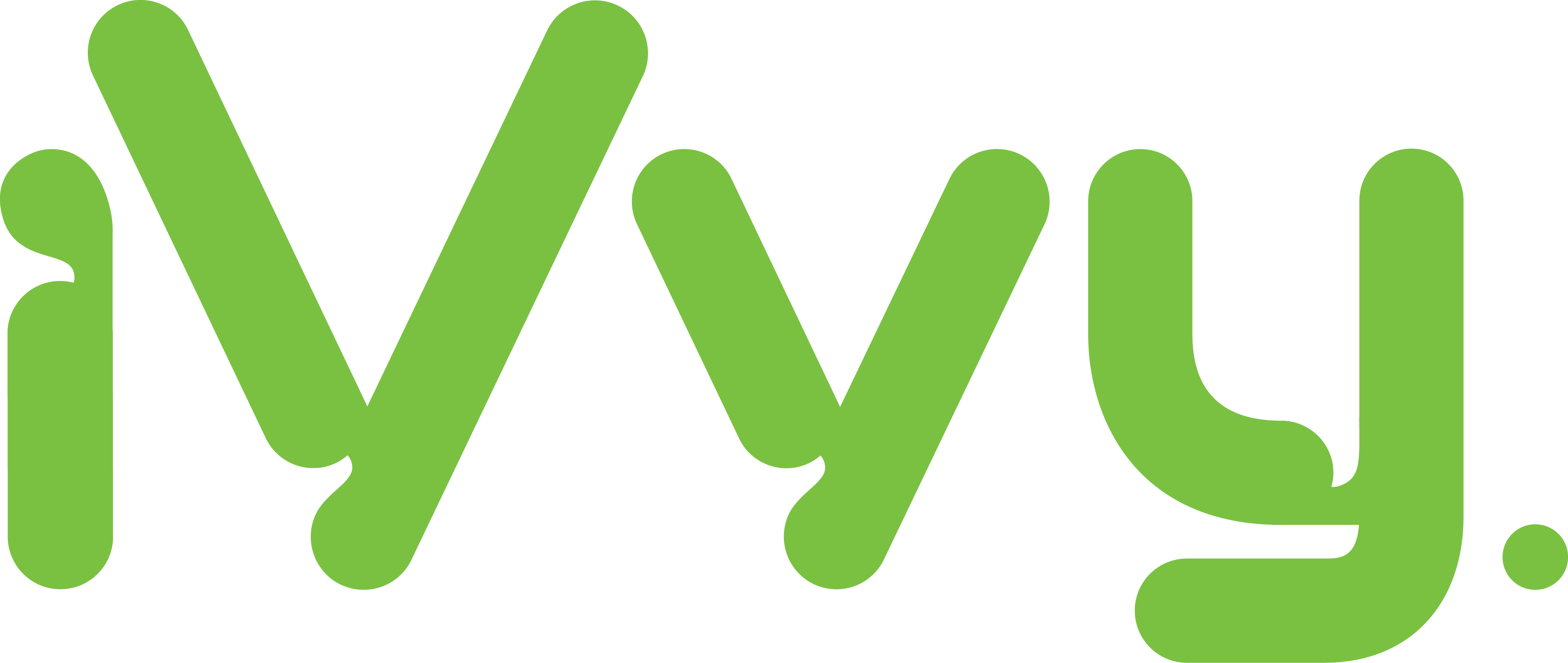The image depicts a series of letters forming what seems to be a brand name or logo on a solid white background. The characters are in a vibrant light green, bubble-style typography with rounded, non-flat edges. Positioned from left to right, the letters are I, V, V, Y, followed by a period. The lowercase "i" stands with an attached dot, which merges into the stem. The first 'V' is larger than the second 'V'. Both V's have rounded indentations at their bases, making the distinction between V's and Y's somewhat ambiguous. The final 'Y' has a distinctive curled-under tail. The letters, especially the V's and Y, have chunks cut out from them, adding a unique, stylized appearance that might make identification challenging at first glance.